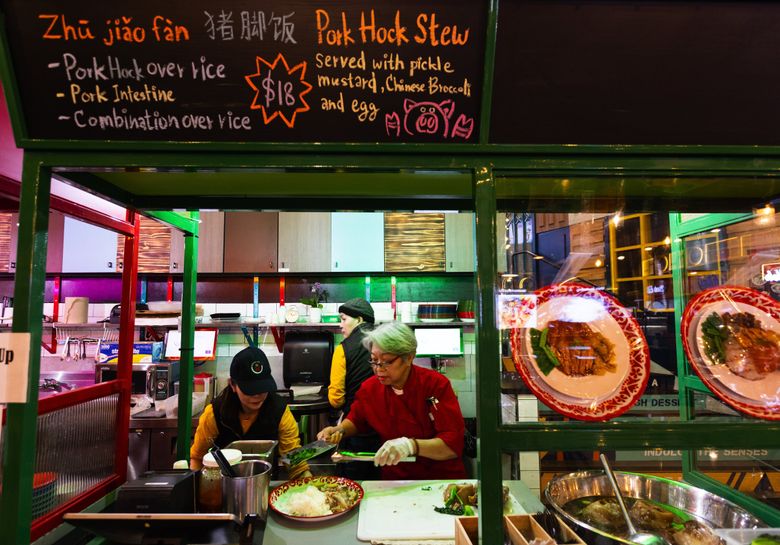In this nighttime photograph of a bustling Asian restaurant or food truck with a green exterior, the central scene is a food ordering window where three people are working. Two women are positioned at the center, with the person on the right donning a red shirt and a white glove on their left hand, and another person on the left in a long-sleeve gold shirt with a black vest. Behind them stands a third person, also wearing a gold shirt, black vest, and a black toboggan, with their back turned to the camera. 

The right side of the image features a large metal circular bowl filled with food, beneath a glass display showcasing sample dishes. Adjacent to this setup is a well-lit chalkboard menu with orange text at the top reading "zhou jiao fan." The menu, written with chalk in various colors, lists items such as "pork hock over rice," "pork intestine," and "combination over rice," all priced at $18. Additional details describe the pork hock stew served with pickled mustard, Chinese broccoli, and egg, accompanied by a whimsical pink drawing of a pig. Plates of prepared food and bowls of cooking ingredients can be seen inside the kitchen, enhancing the image of a lively, authentic dining scene.